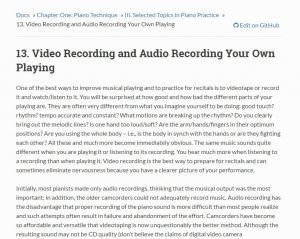The image contains a section of text with a beige background and features the number "13" prominently displayed. The bolded text states "Video Recording and Audio Recording Your Own Playing," suggesting this section's focus. The content is organized into two lengthy paragraphs, which are difficult to read in their entirety. This section appears to be part of "Chapter 1" of a resource titled "Piano Technique," although the blue font makes some of the text challenging to discern. In the upper right corner, there is a prompt in blue that reads "Edit on GitHub," indicating that this document might be a mockup designed for collaborative editing on GitHub. This feature allows users, possibly developers or content reviewers, to submit changes regarding grammar, clarity, or accuracy of the information provided. There are no images in this section—only text.